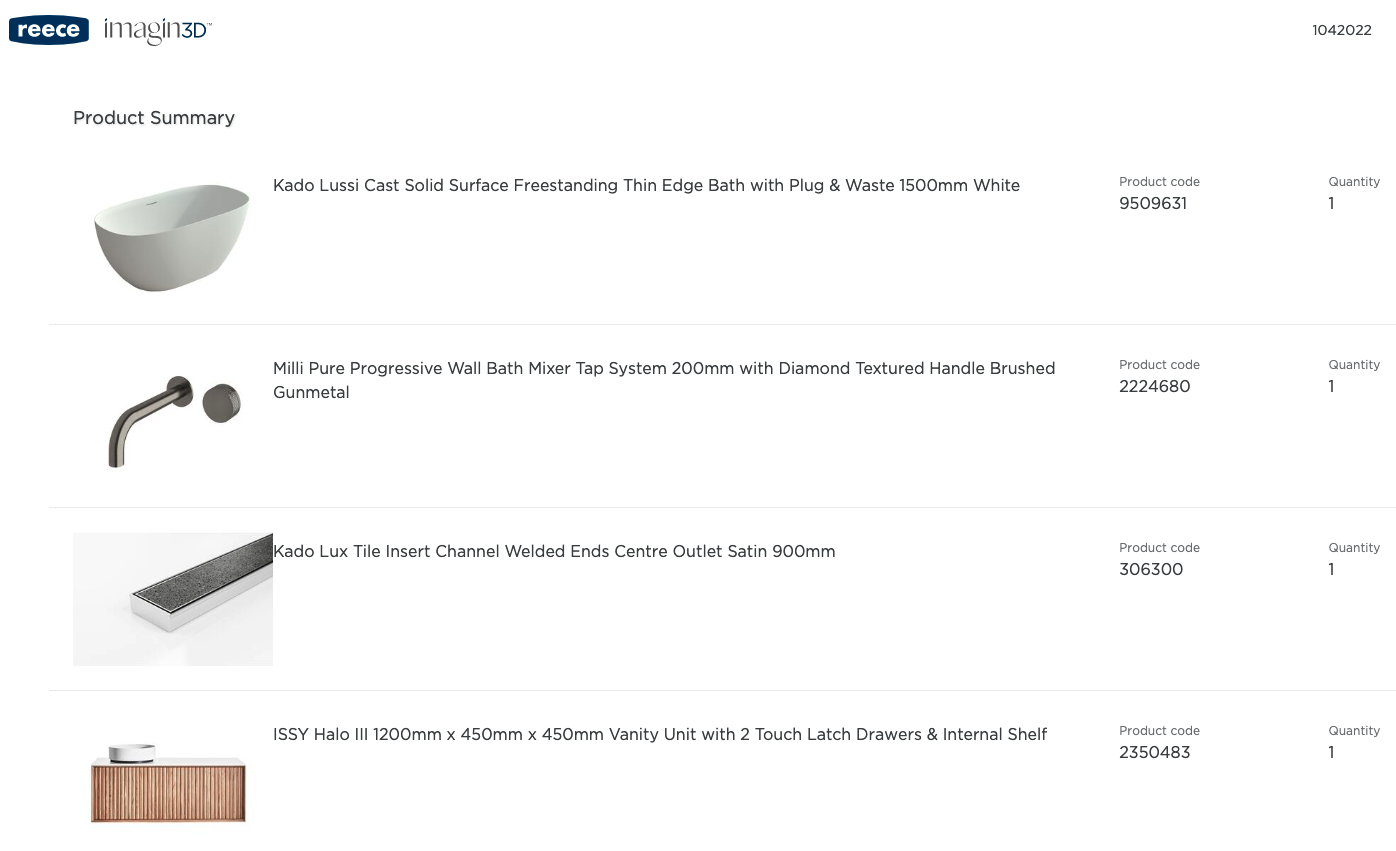The image is a screenshot from the website "Reece Imagined." The logo features "Reece" in a white font inside a dark blue box, next to which the word "Imagined" appears on a white background in a fancier, more stylized font. The letters "I-M-A-G-I-N" are in a grayish color, while the "E" is represented by a stylized "3" and the "D" is capitalized, both in dark blue. In the top right corner, a sequence of numbers "1042022" is visible.

Directly below the website name, the text "Product Summary" appears in black font. Under this header, there is a list of four items, each accompanied by a small preview image to the left. Alongside each image, the product's name, a product code, and the quantity available are listed. Notably, the image does not display any prices or total costs, focusing solely on the product details.